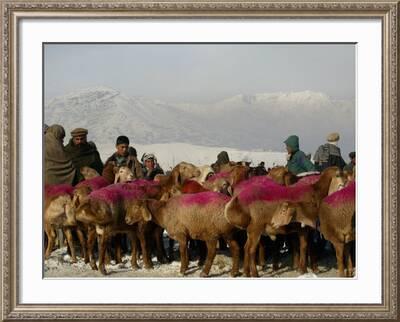The photograph, encased in a solid beige wood frame adorned with engravings and a white inner mat, showcases a vivid color illustration of several shepherds and their sheep. The shepherds, dressed warmly in traditional desert clothing including turbans and cloaks, are tending to a group of sheep with dark, brown coats. Some of the sheep have markings on their backs, which appear to be reddish-pink. The group is set in a snowy landscape, the ground around them mostly clear but with visible snow in the distance. The scene is depicted in a horizontal orientation, with a majestic, snow-capped mountain range and an overcast, gray sky serving as a backdrop. Overall, the image captures the serene yet rugged essence of the shepherds' environment.